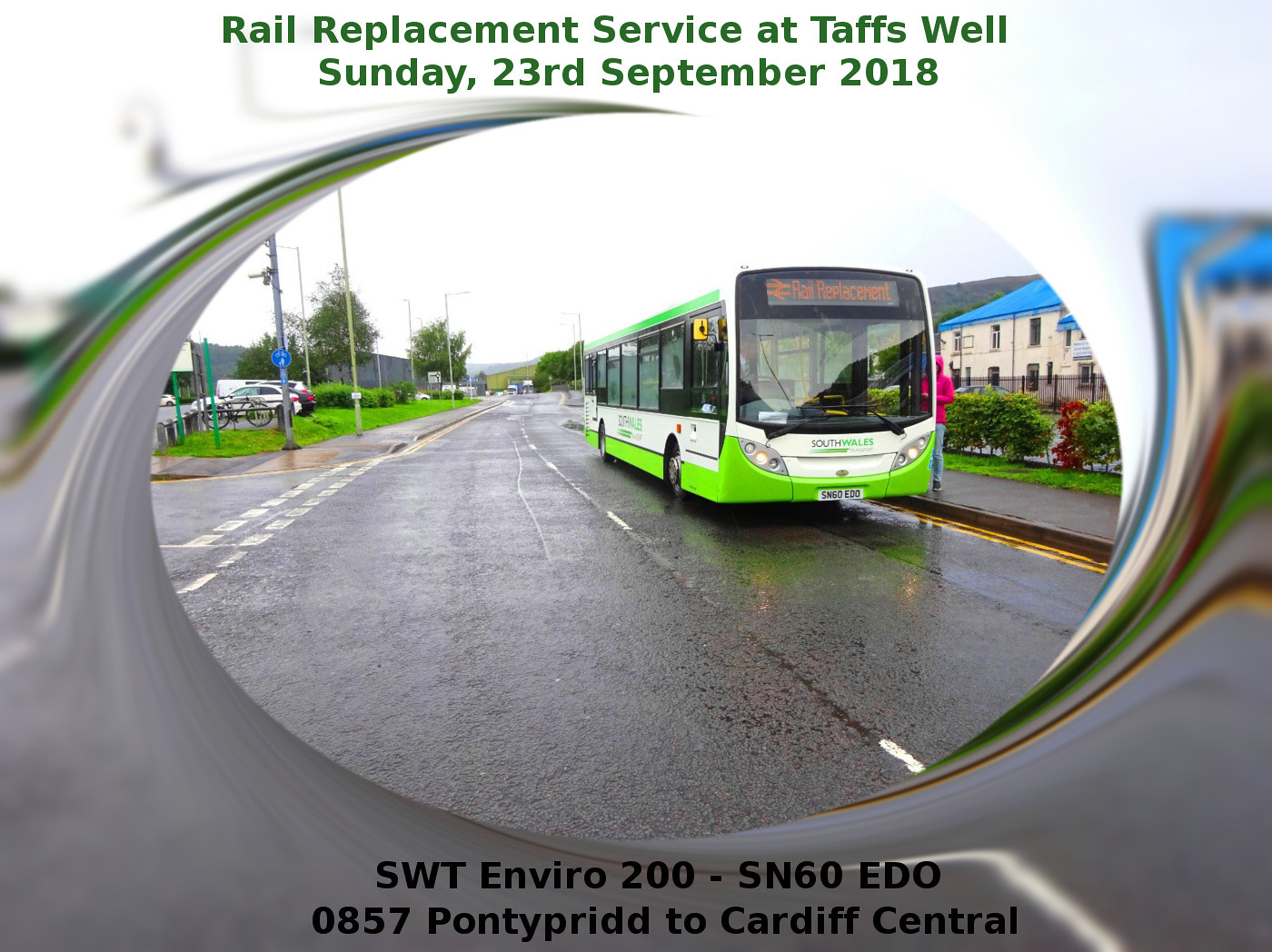This detailed photograph, taken with a fisheye lens that gives the image a swirling, oval border effect, captures a green and white public transportation bus parked on a two-lane street at Taft's Well on Sunday, 23rd September 2018. The text at the top of the image reads "Rail Replacement Service at Taft's Well, Sunday 23rd September 2018" in green letters, while the bottom text states "SWT Enviro 200-SN60EDO" and "0857 Pontypridd to Cardiff Central" in black print. The bus, with "Rail Replacement" and "South Wales" displayed on its front, has the license plate SN60EDO. A person in a pink (or red) hooded sweatshirt and denim jeans is seen boarding the bus on the right. Surrounding the bus on the right side are a sidewalk, grass, bushes, a fence, and a white building with a blue roof. On the left side, the street, another sidewalk, more grass, a fence, a bicycle, some cars, and street lights are visible, along with a blue circular sign hanging from one of the poles in the foreground. The roadway appears wet, adding texture and depth to the scene.